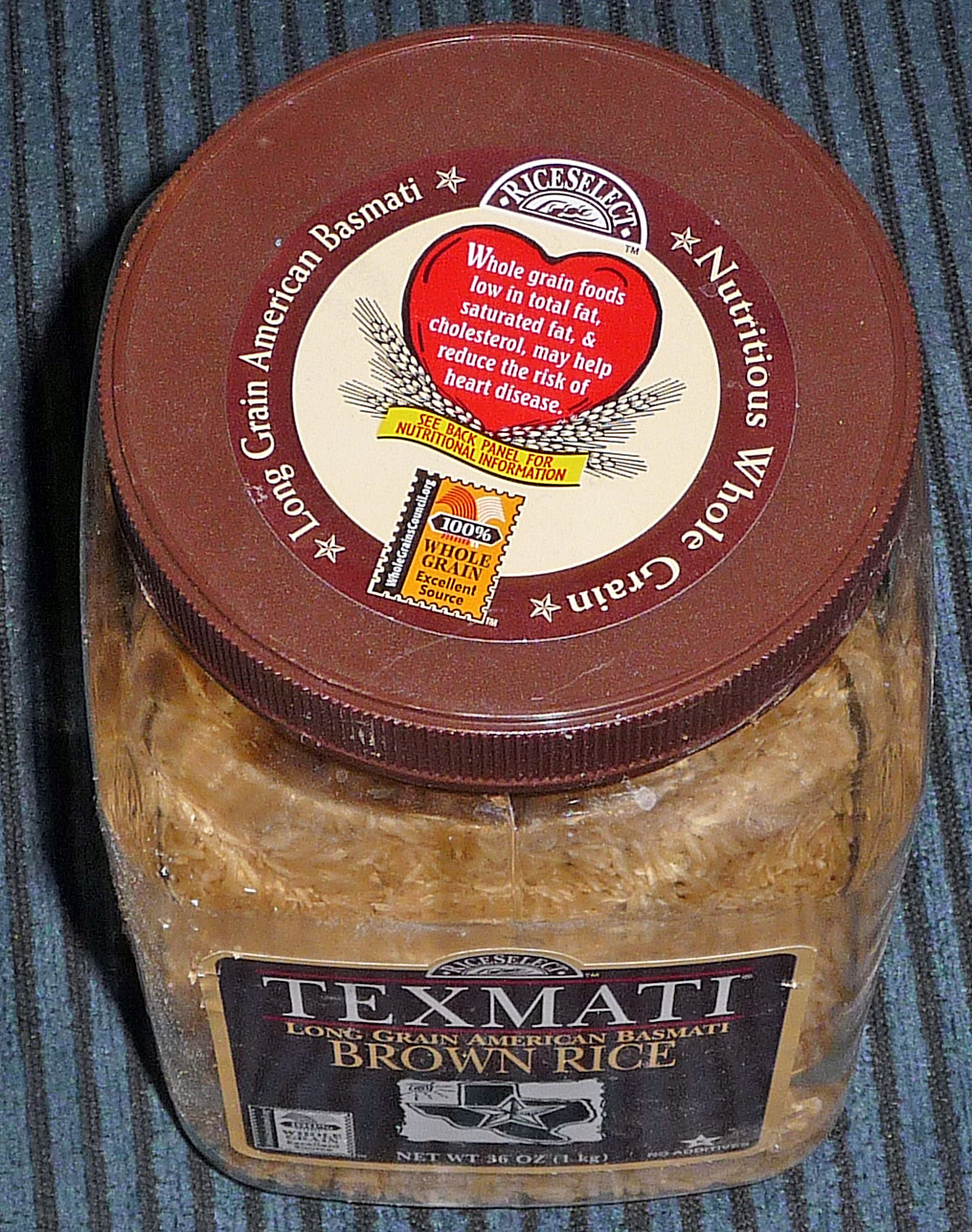This photograph showcases a clear jar filled with basmati rice, positioned on a tea towel with blue and black vertical stripes. The texture and color suggest the tea towel is fuzzy, adding a gentle, cozy background to the image. The jar, which is labeled "TIXMATI, Long Grain American Basmati Brown Rice," features a lid of rich brown color. Prominently displayed, a rectangular white label on the front of the jar illustrates a silhouette of Texas with a star. The perspective of the photograph is from above, allowing a detailed view of the jar's round lid, which bears a sticker. This round sticker repeats the text "LONG GRAIN AMERICAN BASMATI, Nutritious Whole Grain," and includes an emblem of a heart accompanied by wheat or rice stalks beneath it, suggestive of the wholesome and nutritious nature of the rice contained within.